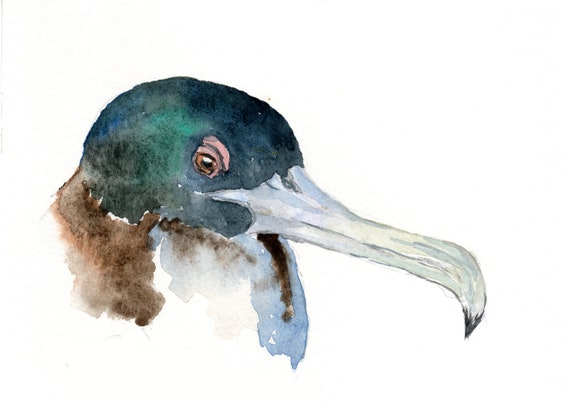A detailed watercolor painting depicts the close-up head of a bird, likely a waterfowl, inside a barely visible, almost invisible, rectangle where the left and right sides seem shorter than the top and bottom. The border is faintly implied, with a pale blue vertical line on the upper left that fades downward. The bird's head reflects a shiny, greenish-black hue that transitions into black at the front, with a tinge of blue at the lower back. The green deepens towards the upper back and right shoulder before easing into brown, which then fades into white and blue as it moves rightward. The bird's eye, located on the right side of its head, is intricately detailed with a brown iris and red eyelids, showing realistic reflection and a vivid focus directed somewhat towards the viewer.

The bird's bill, extending approximately 8 centimeters outward and downward to the right in a diagonal direction, exhibits shades of blue near the face blending into white, concluding with a black tip. The depiction suggests that light comes from the upper right, highlighting the bill's intricate contours and its integration into the bird's face, giving an impression of depth and three-dimensionality. The beak itself curves down at the end and points slightly to the left. Below the head, the image blurs out, with a mixture of blue, white, and a prominent brown streak running down, hinting at either an open beak or the beginning of the bird's neck, but leaving the rest to the viewer's imagination. Overall, the painting combines realistic traits with artistic freedom, potentially inspired by nature or a photograph.